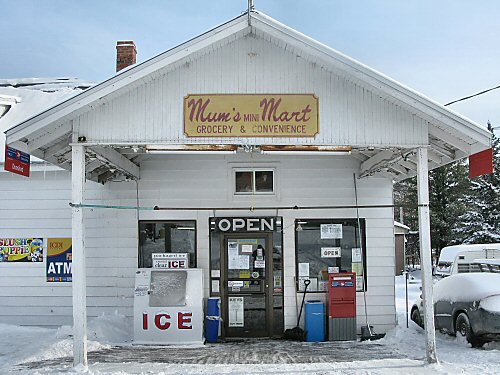In this color photograph, we see a quaint scene featuring a snow-covered mini convenience store. The store is housed in a white, wooden, one-story building that resembles a house, complete with an angled, gabled roof and a brick chimney. Above the glass door entrance, framed by two square windows, is a mustard-colored sign with prominent red letters reading "MUM's Mini Mart." Subtext on the sign indicates the store offers "Grocery and Convenience." Just above the door, another sign in white letters on a black background declares "OPEN."

To the left of the doorway stands a white icebox with the word "ICE" emblazoned in red letters, while on the right, a blue and red container along with a snow shovel are visible. In front of the store, snow blankets the ground and covers several parked cars. In the distance, snow-covered pine trees enhance the wintry ambiance, and a nearby garage can be seen. The scene is set against a backdrop of a blue sky with scattered clouds, completing this picturesque, wintry depiction of MUM's Mini Mart.